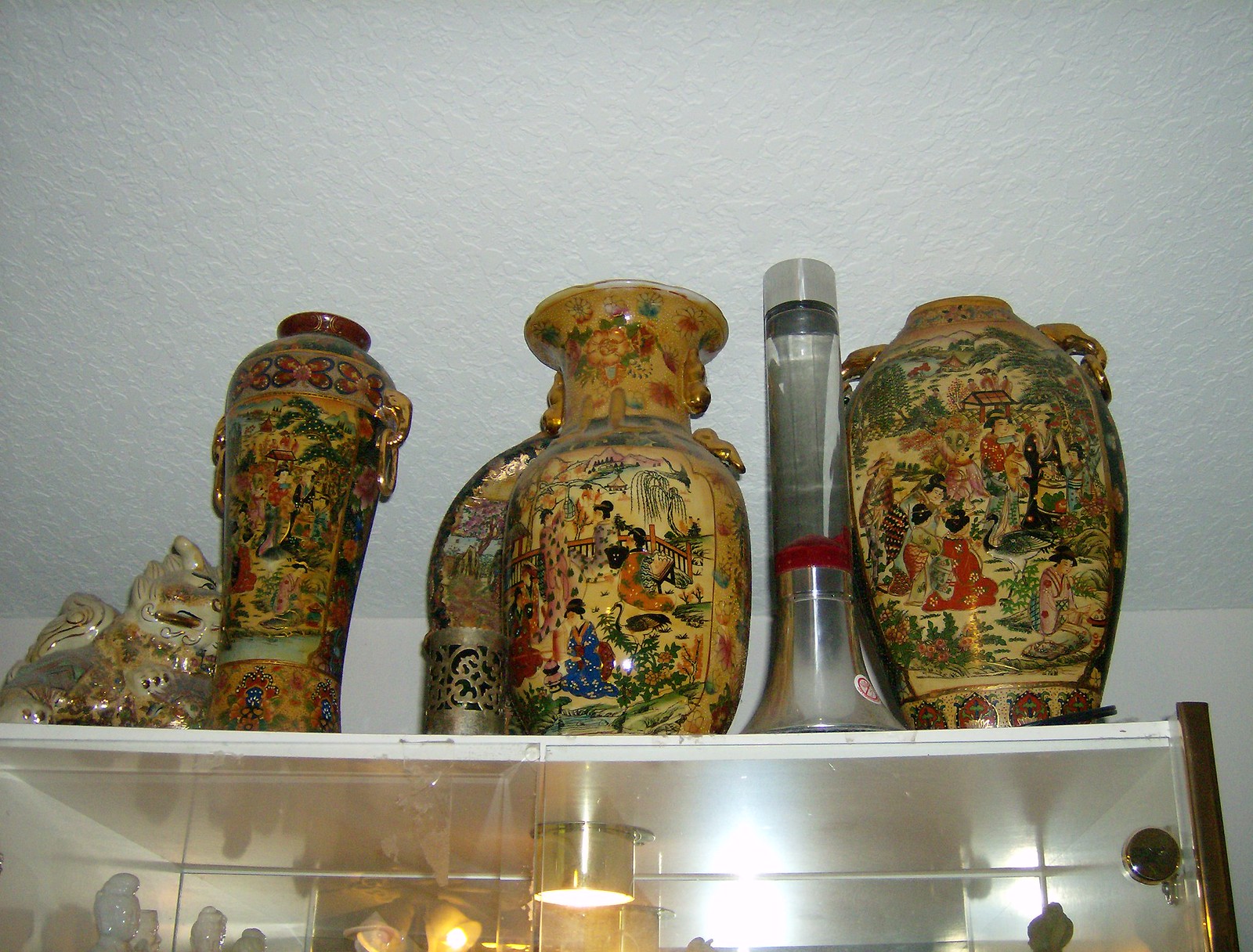This high-quality photograph captures an ornate display atop a cabinet, featuring four vases and an assortment of decorations. Dominating the scene, the vases are adorned with intricate artwork depicting various figures, predominantly Asian women, engaged in activities such as bowing and praying within what appears to be a village setting. The designs include vivid colors—yellows, blues, oranges, and reds—and show detailed elements like bushes, trees, fences, lakes, and waterfalls, suggestive of Asian landscapes. Each vase varies in shape and size: the one on the far left is slender, the central one tapers elegantly from a round base, and the rightmost vase is distinguished by its large oval form. Between the central and right vases, there is a smaller, unidentifiable object that appears to be plastic. Additionally, a figurine of a cat can be seen on the far left, contributing to the eclectic yet harmonious arrangement.